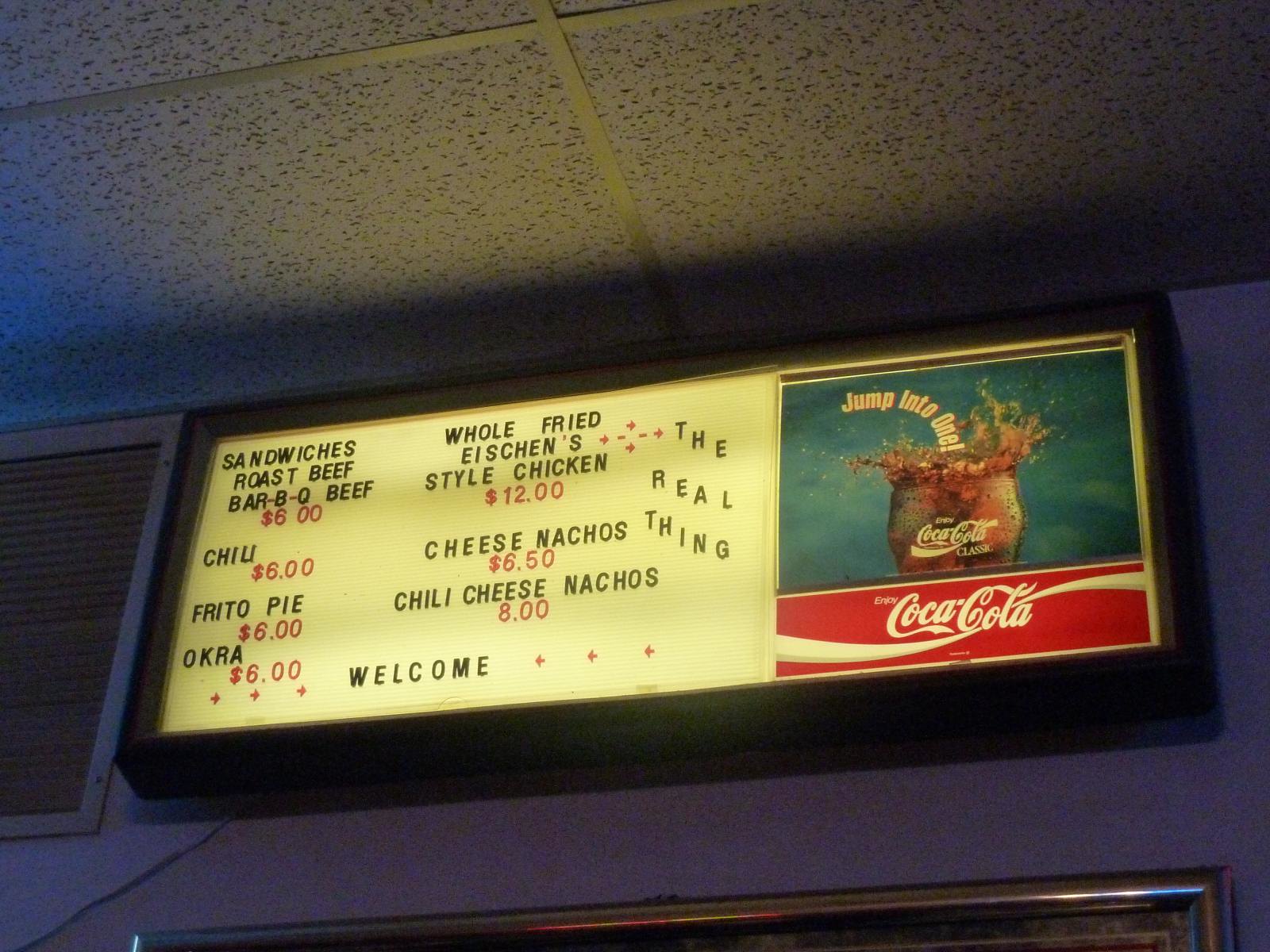The image portrays a close-up photo of a restaurant menu board mounted near the ceiling on the wall. The menu lists various items, with offerings including sandwiches, roast beef, and BBQ beef, each priced at $6. Other menu selections are chili for $6, Frito Pie for $6, and okra also for $6. Additionally, they offer a whole fried Asian-style chicken for $12, cheese nachos for $6.50, and chili cheese nachos for $8. Along the side of the menu, the phrase "The Real Thing" is written in a slanted font, descending vertically. At the bottom of the sign, the word "Welcome" is displayed, flanked by red star shapes on both sides. The menu items are written in black text, while the prices are highlighted in red. To the right of the menu, there is a prominent Coca-Cola logo set against a red rectangular background. Above the Coca-Cola logo is an image of a glass of Coca-Cola, featuring the slogan "Jump into One" in a white, curved font, accompanied by a splash of soda for emphasis.